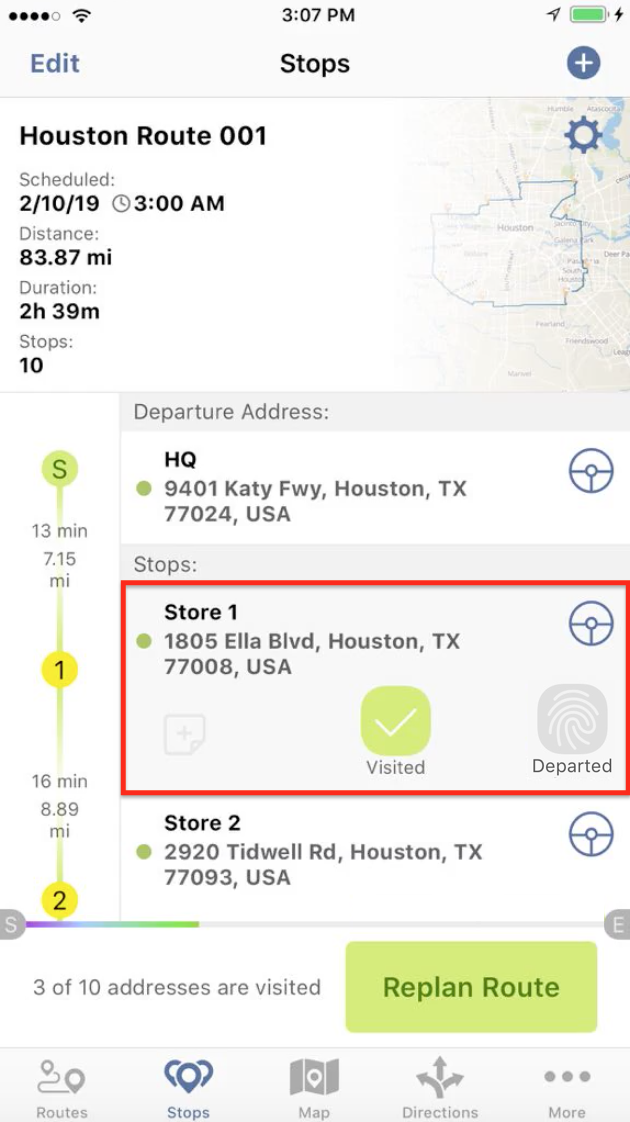The image displays a mobile screen showcasing a navigation and logistics application. At the top center, the time is displayed as 3:07 PM, flanked by the battery icon on the right and signal strength and Wi-Fi indicators on the left. Below this, there is an "Edit" button and a circular icon with a plus sign.

The main section of the screen details a route titled "Houston Route 001" with a schedule date of 02/10/19 at 3:00 AM. The route encompasses a total distance of 83.87 miles and an estimated duration of 2 hours and 39 minutes, encompassing 10 stops. A partially visible map outlines the Houston area.

The departure address is listed as HQ, 9401 Katy Freeway, Houston, Texas, 77024, USA, accompanied by a circle icon with a steering wheel. 

The first stop, labeled as Store 1, is located at 1805 Ella Boulevard, Houston, Texas, 77008, USA, identified by its circle steering wheel icon. Below the address, there are indicators showing "Visited" and "Departed" statuses. 

The second stop, Store 2, is at 2920 Tidwell Road, Houston, Texas, 77093, USA, marked by a green circle with an 'S'. The route specifics indicate a 13-minute duration covering 7.15 miles to a yellow circle marked '1', then a 16-minute duration covering 8.89 miles to a circle marked '2'.

Near the bottom of the screen, it shows that 3 out of 10 addresses have been visited with an option to "Replan Route." Lastly, at the very bottom, icons for "Routes," "Stops," "Map," "Direction," and "More" are displayed, providing additional functionalities.